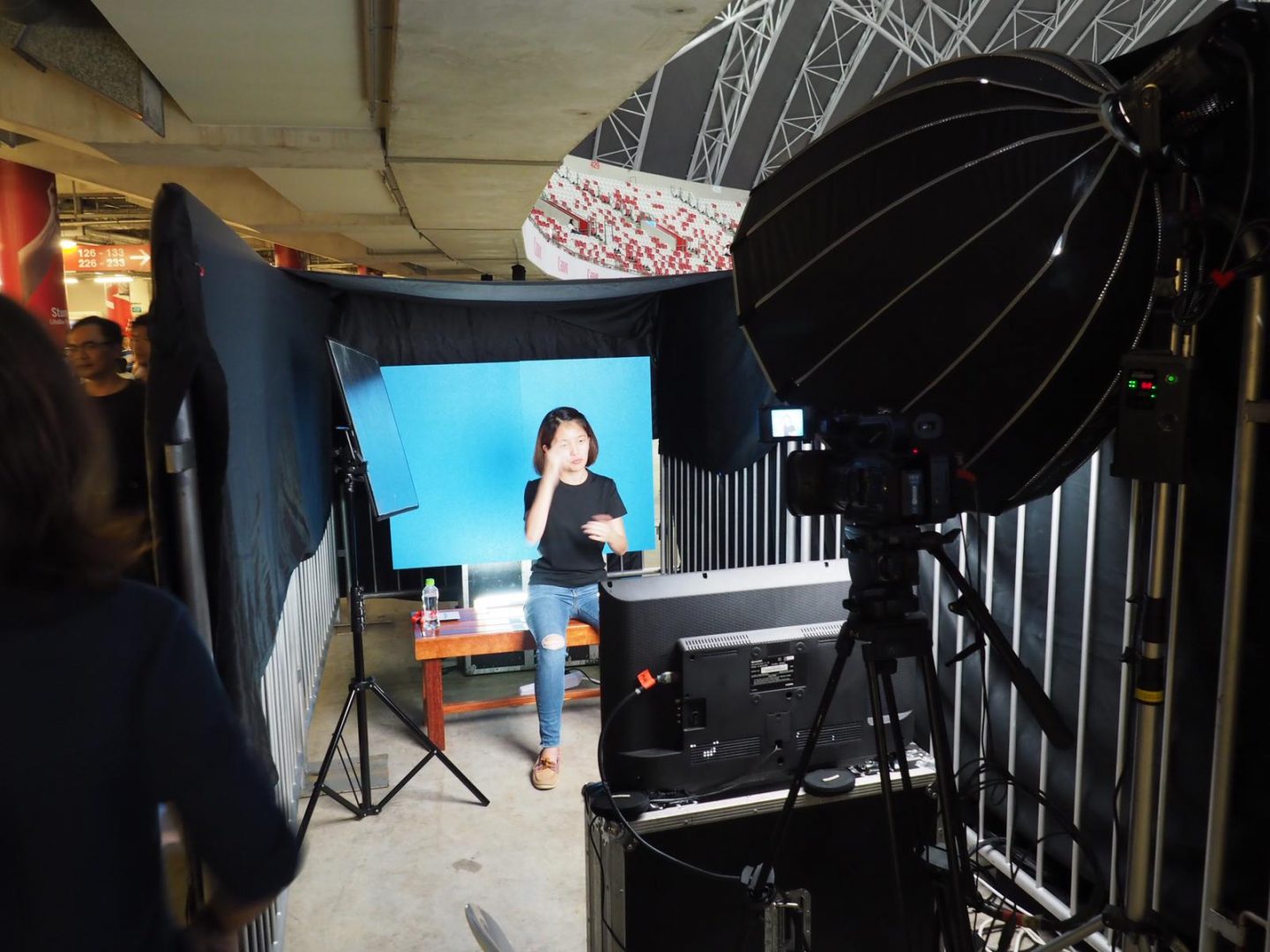This horizontally oriented color photograph captures an intricate photography studio setup within a larger venue. Positioned in the lower section of the frame is the photography studio, encircled by grandstands or audience seating situated above. To the left, a hallway is visible where people are walking, indicating a bustling atmosphere outside the studio. The ceiling above the studio setup is notably low.

Central to the composition is a woman sitting on a wooden bench, posed against a blue backdrop. She is dressed in a black t-shirt and jeans with a noticeable hole in the right knee. Her right hand is elegantly touching her right eyebrow. To her left, a screen is mounted on a tripod, suggesting it's a reflector or diffuser for lighting.

The right side of the image reveals the back of the studio equipment, encompassing a screen atop a musical equipment case, which could be used for previewing shots. A large spotlight with a curved lampshade is also visible from the rear, enhancing the lighting on the subject. Additionally, a camera on a tripod with a small preview screen is capturing the woman's pose on the bench. The overall setup and the bright spotlight focused on the woman emphasize that this is a professional photo shoot in progress.